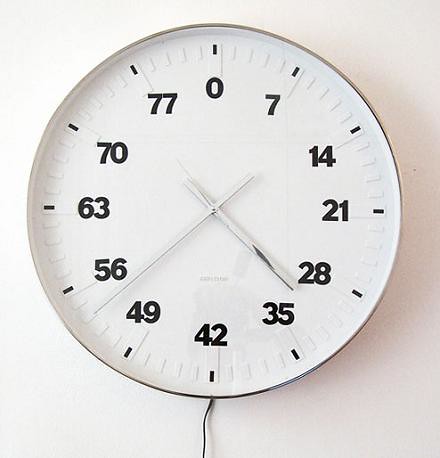The image depicts a uniquely designed clock with a white face and white hands, omitting the second hand and featuring only the minute and hour hands. Instead of the conventional numbering system from 1 to 12, this clock face is marked by multiples of 7. Starting from the top, the numbers sequentially increase by 7: positioned at what would normally be the 1 o'clock spot is the number 7, followed by 14 at the 2 o'clock position, 21 at 3 o'clock, and so on, until 77 replaces the 11 o'clock spot, and finally, the 12 o'clock position is marked with 0. The clock face also displays black dots at each hour position for additional clarity. Currently, the small hour hand points towards 30, while the larger minute hand is directed at 54. Analyzing the conventional time, this positioning corresponds to 4:38.